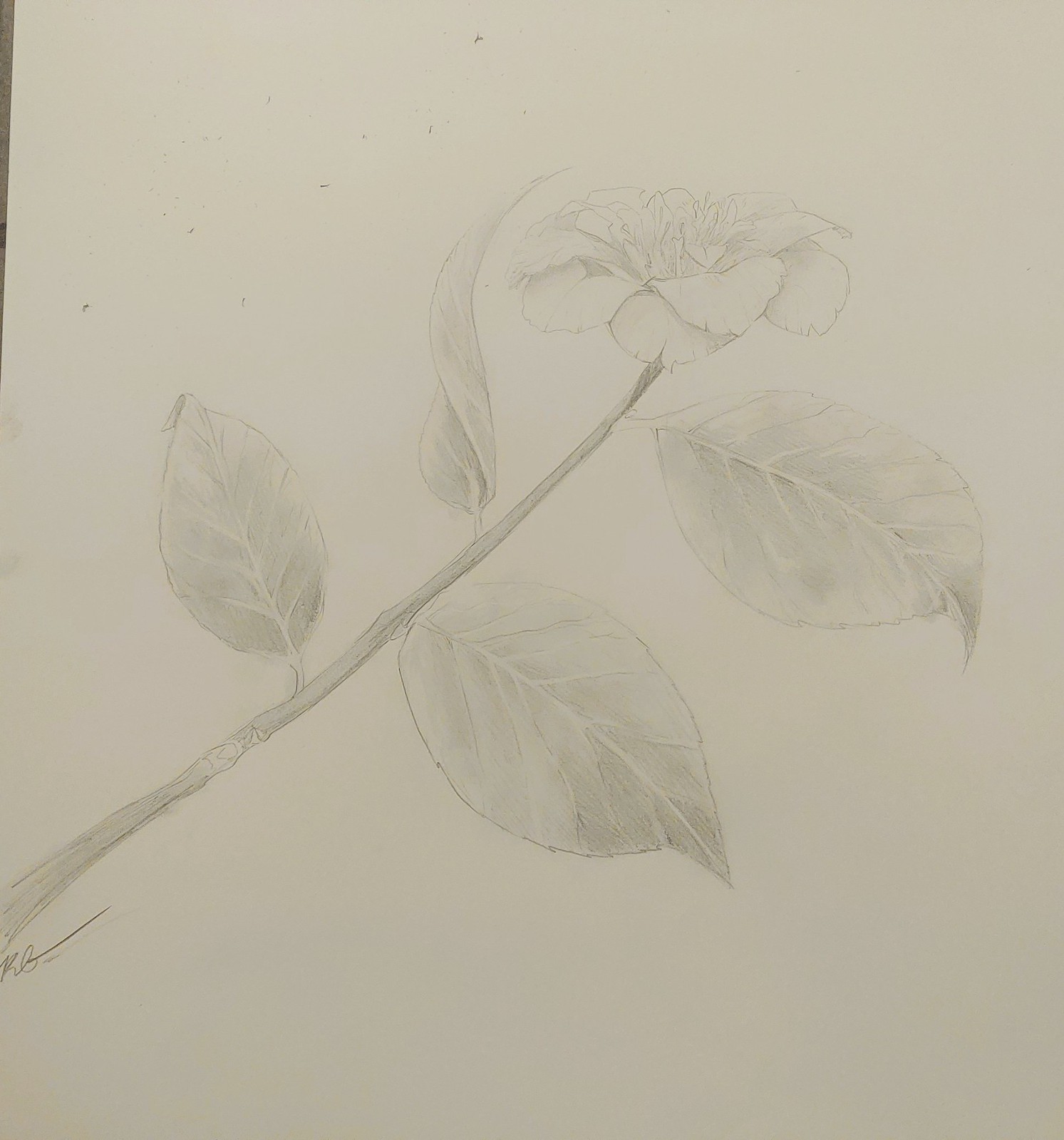This detailed pencil drawing, set against a cream-colored piece of paper, showcases an intricate flower design. Nestled primarily in the middle of the paper, the flower's long stem extends from the bottom left corner, diagonally rising about three-quarters of the way towards the upper right. The stem culminates in a beautifully detailed bloom that points gracefully upwards in the top right corner. The flower is adorned with four delicately drawn leaves, two on each side of the stem. The top-left leaf gently curves sideways, creating a subtle dynamic contrast to the other three leaves, which all point upward in unison with the flower. In the very top left corner of the image, a glimpse of a room suggests the drawing was photographed rather than digitally scanned, adding an element of context to this lovely botanical artwork.